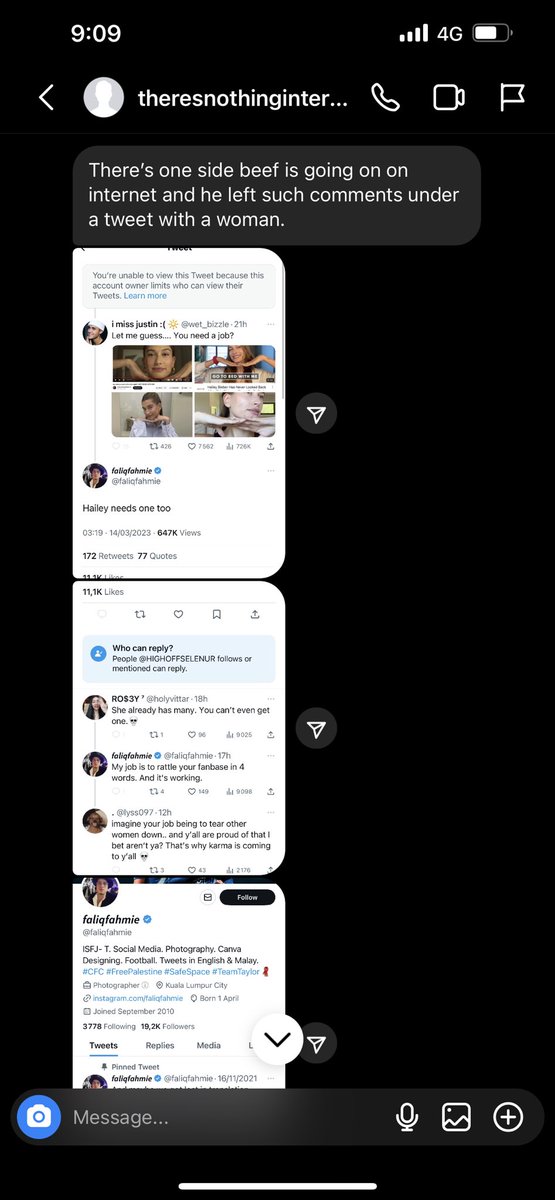The image is a vertically-oriented snapshot taken from a cellphone screen with a black background. At the top left corner, the time is displayed as '9:09'. Opposite on the top right, the signal strength is indicated with four bars, marked '4G', and a battery icon showing approximately 75% charge.

Below this status bar, on the left-hand side, there is a back arrow icon, followed by a small white circle containing a head icon. Next to it, text reads, "There's nothing enter..." Ellipsis follows this text. Moving right, there are icons for a phone camera and a flag symbol.

Just below this, a text box is visible displaying the message: "There's one side beef is going on on the internet and he left such comments under a tweet with a woman." Below this text box, there are three small white boxes containing text that is too small to read clearly from the snapshot. These boxes seem to contain conversations on Twitter, each marked by arrows pointing to the upper right corner.

At the bottom of the screenshot, a white circle with a downward-pointing black arrow is present. Adjacent to this, a dialogue box contains a blue circle with a camera icon labeled 'Message'. To the right of this, there are icons showing a microphone, a landscape, and a plus symbol.